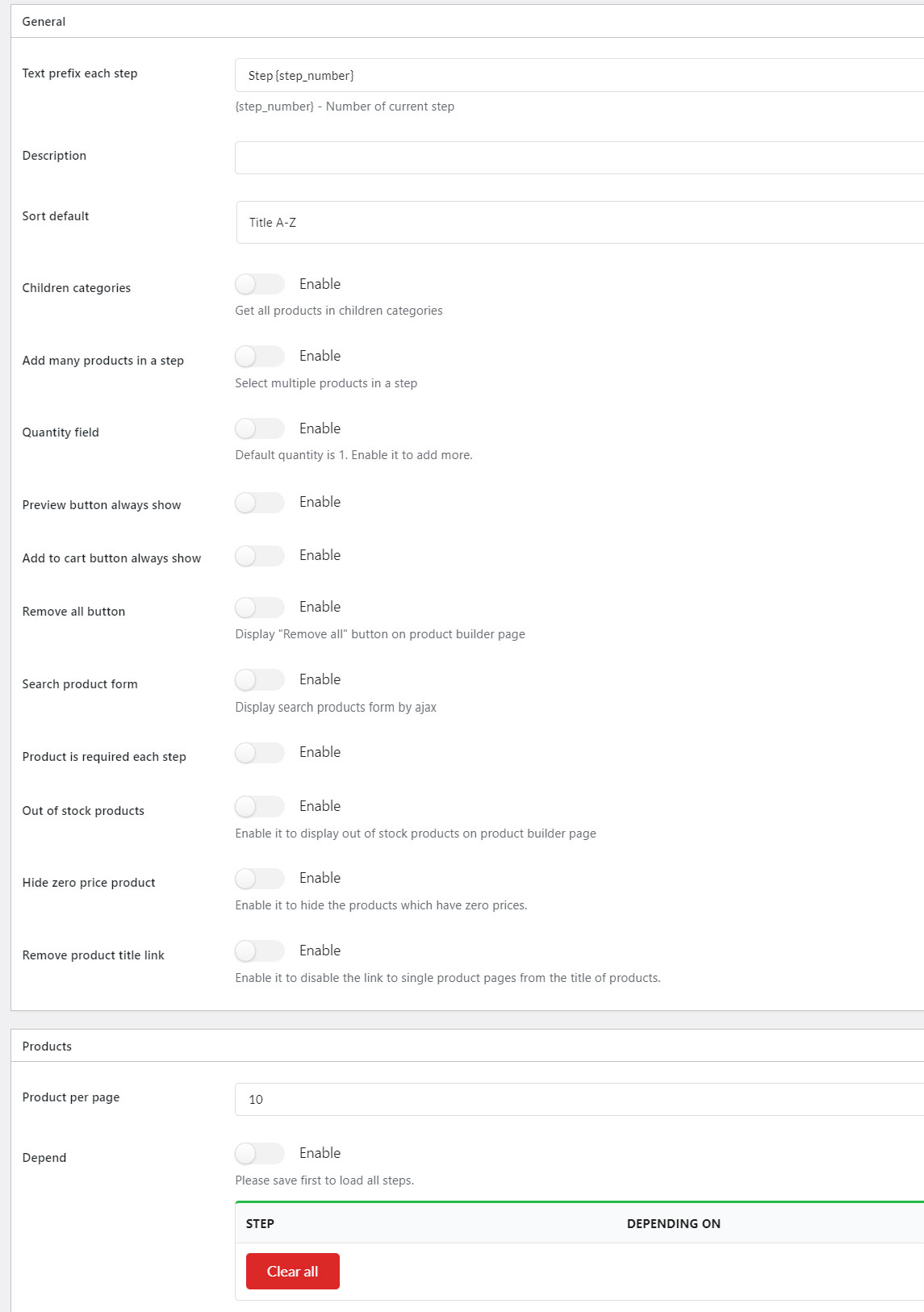In the provided image, we see a detailed interface of a menu, predominantly with a white background and black text for all the options and buttons. At the top of the page is a general bar, followed by the text "Prefix Each Step". Below this, there is a description bar, and then a section labeled "Sort Default" with a space allowing input for titles, sorted alphabetically from A to Z. 

Following that, we notice options for children categories and an adjacent button to enable or disable these categories. Further down, there’s an “Add Many Products in a Step” option alongside a quantity field bar. There are buttons for displaying a preview and “Add to Cart,” consistently set to "always show". The interface also features a “Remove All” button and a “Search Product” form. 

Options are provided to mark products as required for each step, hide out-of-stock products, hide zero-price products, and remove the product title link—each of these has an enable option to show the respective results.

Below these settings, there is a section dedicated to product display, allowing users to set the number of products per page, which is currently set to 10. Additionally, there is an enable button for the "Depend" option, and beneath this, another box labeled "Step," which gives options based on dependencies, along with a button to clear all settings.

The overall layout maintains a clean and orderly design, with a white background that contrasts with the black text, ensuring readability of the various options and features.